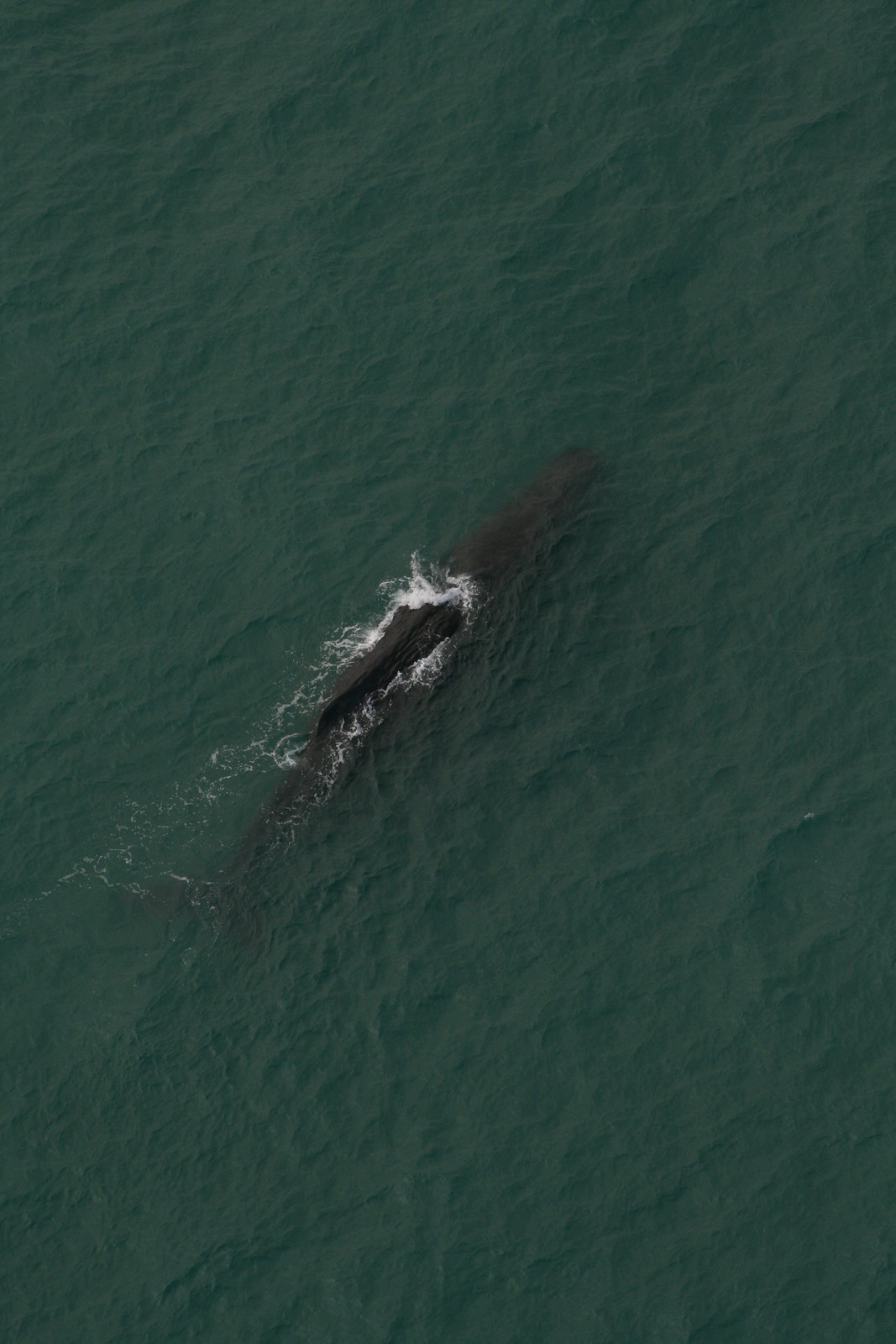An overhead photograph reveals a large sea creature, potentially a whale or a massive fish, swimming in a rich, forest green ocean with hints of blue. The animal's dark charcoal gray body, partially submerged and partially exposed, creates a dynamic splash and white water surrounding its fin as it moves through the rippling sea, indicating a breezy day. The high-altitude perspective, likely taken from a helicopter, captures the scene with clarity in daytime, suggesting the creature's significant size and weight—possibly hundreds of pounds. This impressive aquatic display makes the viewer feel the vastness and wild beauty of the open ocean.